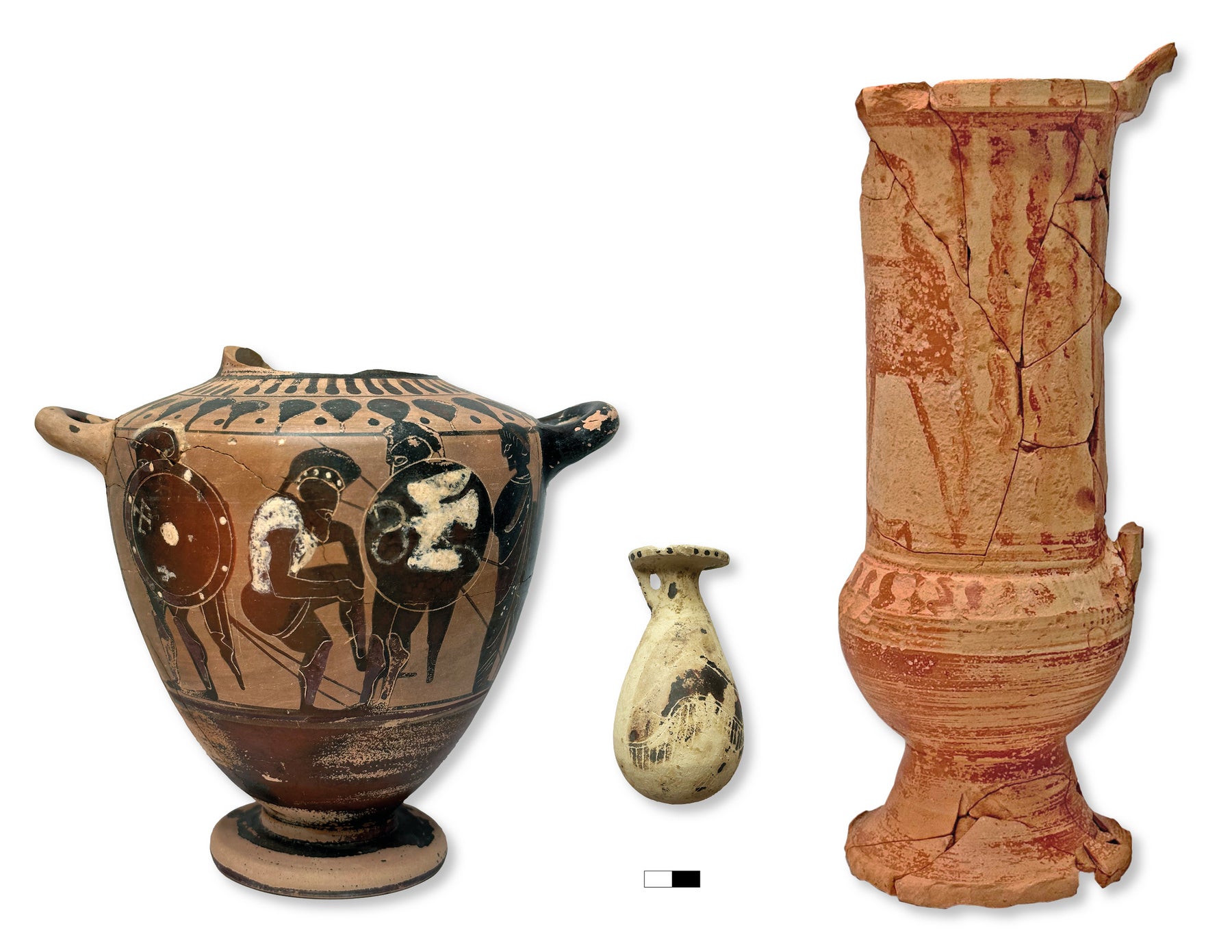This image features three distinct pieces of ancient pottery, presented against a white background in a landscape orientation. On the left is a wide and squat vase with two round handles. The top of the vase is chipped, revealing a clear, broken edge. The vase is adorned with intricate illustrations of warriors equipped with ornate helmets and shields. One shield has an hourglass shape with a dove motif, while another is rusty-colored with dots and insignias. A central warrior, appearing to wear a fur top or vest, is depicted with a raised leg as if dancing. The vase boasts a color palette of light browns, blacks, and rust hues. 

In the middle, there is a smaller vase, markedly petite in comparison to the others. It features a single handle on the left side and a flat top that raises questions about whether it is open or solid. This piece is mostly pearly egg-colored with black and gray splotches, giving it an aged appearance. The finish is notably worn off in certain areas.

On the right stands a tall, cylindrical vase. This piece, once likely equipped with a handle on the right side, shows visible cracks and reassembly marks where it has been repaired. The vase is primarily in muted orange and red tones with a slightly off-taupe hue. It has a rounded bottom part leading up to what appears to be a more fluted base structure.

These pieces illustrate the intricate and varied craftsmanship of ancient pottery, with detailed and evocative designs that evoke a glimpse into the artistic and functional dimensions of their time.